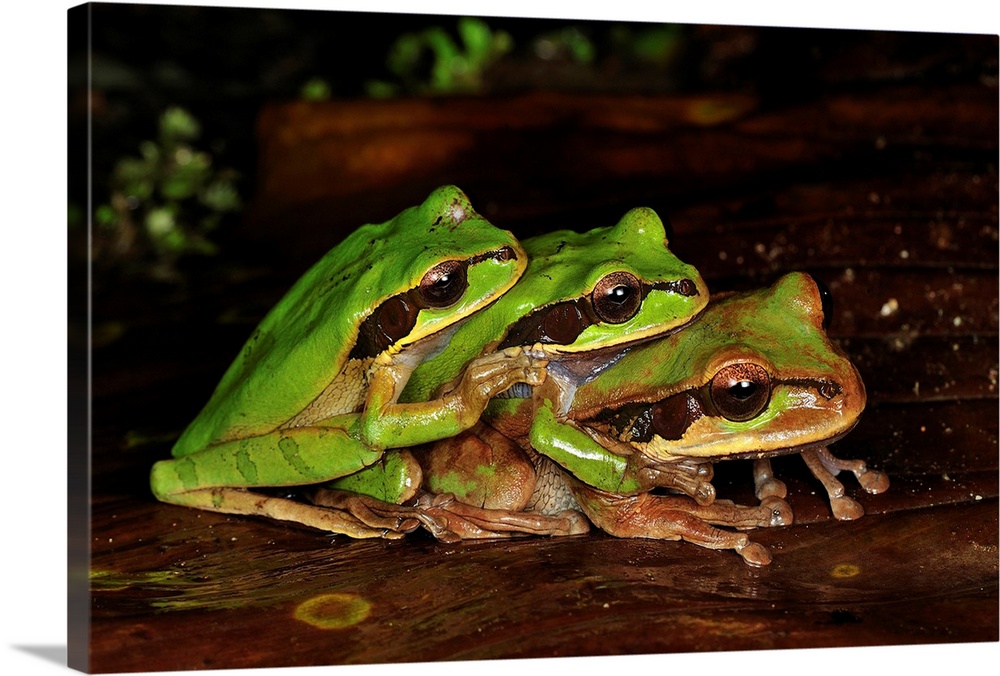This image shows a detailed canvas print featuring three vibrant green frogs huddled together on a log. The frogs, speckled with brown and adorned with a stripe running from their nostrils across their eyes to their front legs, are arranged in a leapfrog-like position, with each frog resting on the back of the one below it. The log they are perched on appears wet, suggesting a natural, damp habitat. Behind them, the background is blurred with hints of greenery and additional wood, creating a dark, muted atmosphere that contrasts with the bright hues of the frogs. The canvas itself is displayed at an angle, allowing for a view of its thickness and texture. Notably, the lowest frog is partially covered in mud and dirt, adding a touch of realism to the scene.